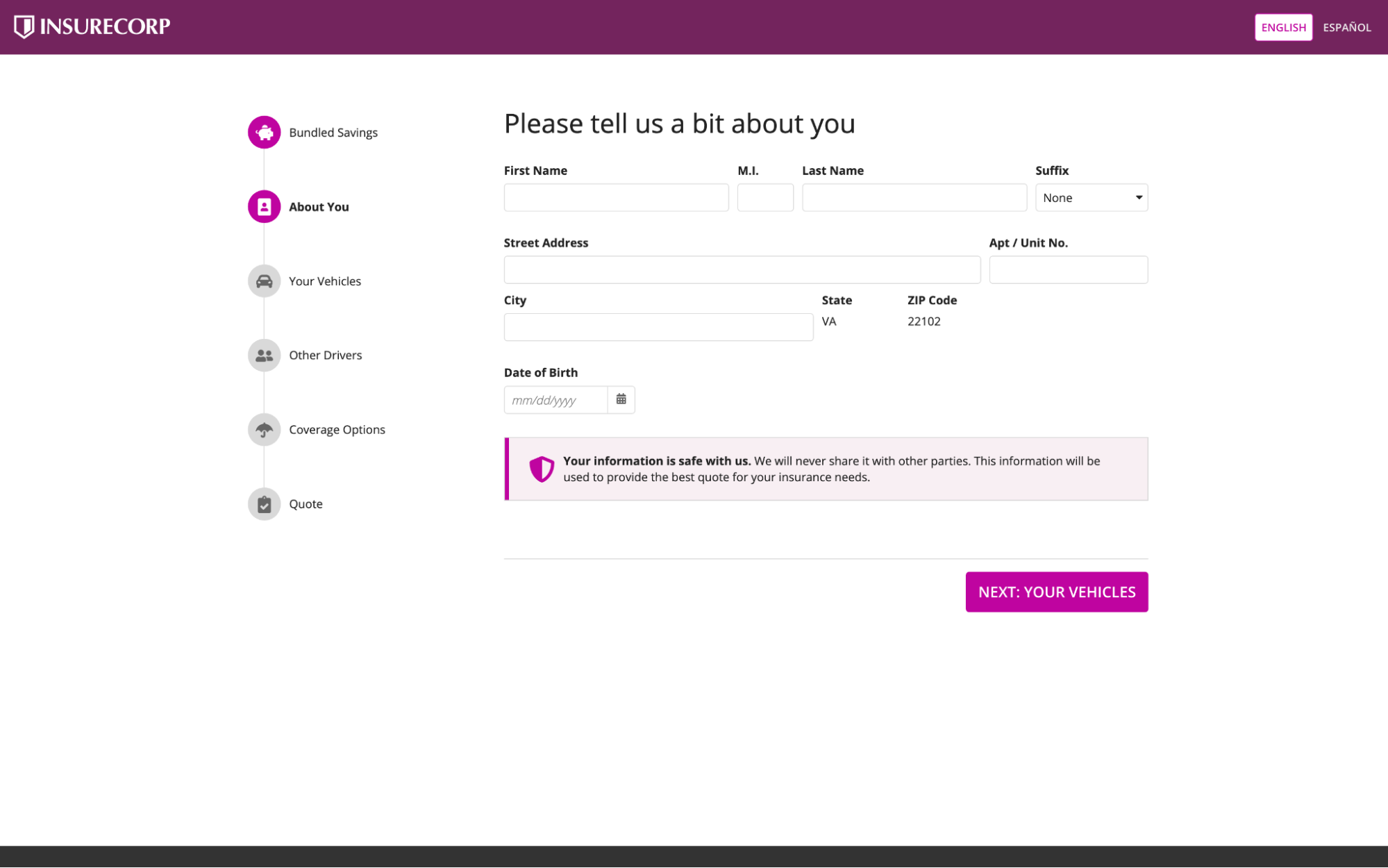The image is a screenshot of a web form on the InsureCorp website, designed for the purpose of gathering user information for insurance quotes.

At the top of the form, there is a maroon-purple band featuring a half-white shield logo on the left, accompanied by the text "InsureCorp." On the right side of this band, the language is set to English, with an option to switch to Spanish.

On the left-hand side of the interface, a vertical stack of round icons helps to navigate different sections of the form. The currently active section, "About You," is highlighted with a maroon outline. The other sections—"Your Vehicles," "Other Drivers," "Coverage Options," and "Quotes"—are grayed out, indicating they have yet to be filled out.

The main portion of the form asks the user for personal information. The fields include:
- First Name
- Middle Initial
- Last Name
- Suffix (with "None" pre-selected)
- Street Address
- Apartment/Unit Number
- City
- State (pre-filled with "VA")
- Zip Code (filled with "22102")
- Date of Birth (with separate fields for Month, Day, and Year, and an accompanying calendar icon)

Below these fields, a light gray rectangle contains a security reassurance message next to the same maroon shield logo. The black text reads: "Your information is safe with us. We will never share it with other parties. This information will be used to provide the best quote for your insurance needs."

A thin horizontal gray line separates this message from the next section of the form. At the bottom right corner, there is a maroon button with white text that says, "Next: Your Vehicles."